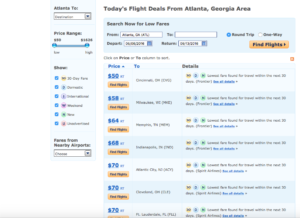The image appears to be a screenshot from a travel website focused on offering flight deals from the Atlanta, Georgia area. At the top of the image, there's a clear header stating "Today's Flight Deals from Atlanta, Georgia." The website interface includes options for selecting roundtrip tickets, which is currently checked, while the one-way option is not selected. 

There are sections within the interface for entering departure and return dates, surrounded by rectangular boxes labeled "Find Flights." The text inside these boxes and other details about departure and return dates are blurry and difficult to read. 

Price ranges are hinted at in the image, although specific numbers are hard to decipher. Lines of different prices suggest a range of deals, with unclear listings such as $58, $64, $68, $70, and $70, possibly representing different flight options or dates. These price listings come from nearby airports and are highlighted in various colors, including yellow, blue, and black.

The background of the image is mostly white, contributing to its pixelated and blurry appearance, making it evident that the screenshot was taken from a website specializing in flight deal searches. Despite the poor image quality, it's clear that the user intended to highlight fluctuating prices and available flight options.